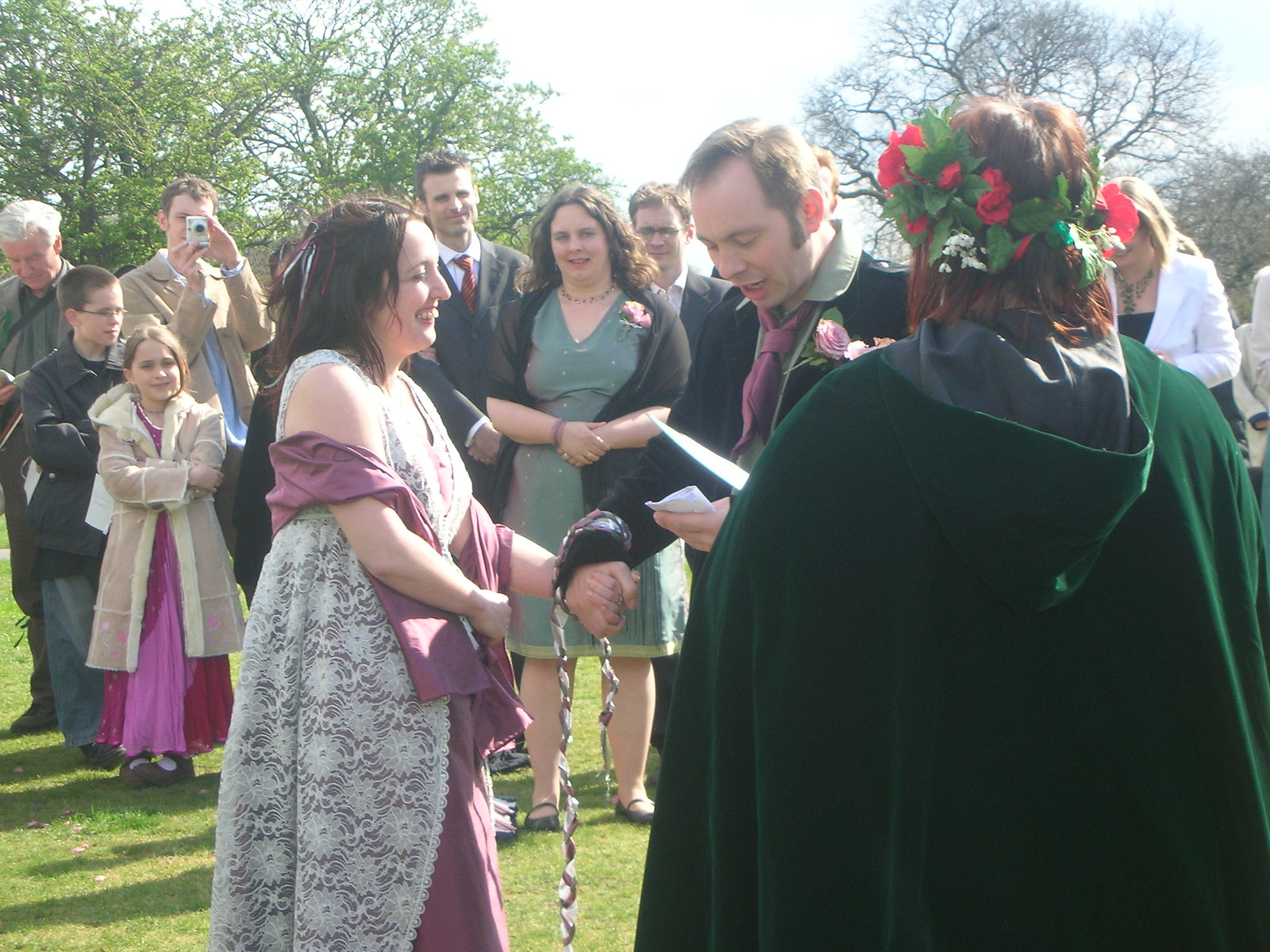In this picturesque outdoor wedding ceremony, a bride and groom, both of Caucasian descent, stand at the forefront of a gathered crowd, beneath the overcast sky with the serene backdrop of trees. The bride is elegantly adorned in a white lacy dress complemented by a purply-pink, blush-colored gown with dark hair cascading down. The groom, matching her in aesthetic harmony, dons a black tuxedo accentuated by a purple tie, his dark hair neatly styled. They stand with their hands clasped and bound by a purple and white ribbon symbolizing their union. The officiant, a woman dressed in green druidic robes with an elaborate, flowery headdress, stands before them, facing both the couple and the assembly behind, where guests, some taking pictures, watch attentively on the grassy terrain. The groom, holding a piece of paper, addresses his bride, seemingly giving a heartfelt speech, adding to the intimate and slightly renaissance-like ambiance of the scene.